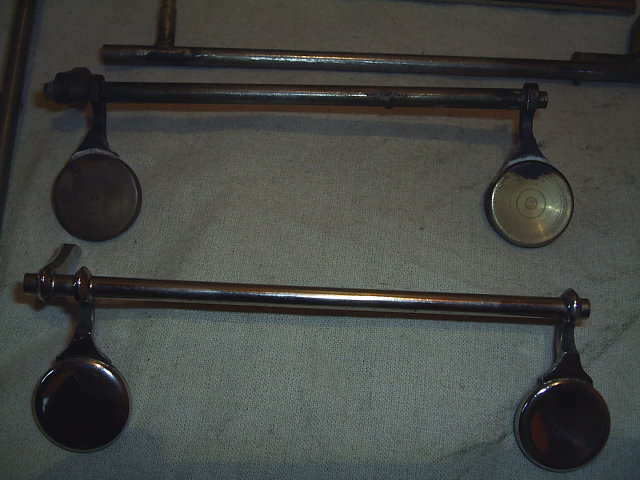This color photo, although darkly lit, captures three old, rusty metal implements laid out on a piece of brown linen cloth. Each implement consists of a horizontal metal bar, heavily tarnished, and attached to it are dish-like structures that resemble small frying pans or shower heads, but without any holes. These circular attachments, more goldish or brass in color, are tarnished and appear to be non-mobile, hanging like pendants from the bars. Each implement casts a shadow on the fabric, adding depth to the image. The topmost and middle implements show different angles of the disc-like attachments, giving the impression that some have necks like frying pans, while others appear flatter, akin to dish pans. The photo gives a detailed look at the aged and rustic texture of both the rods and the circular attachments, emphasizing their antiquated and mysterious nature.